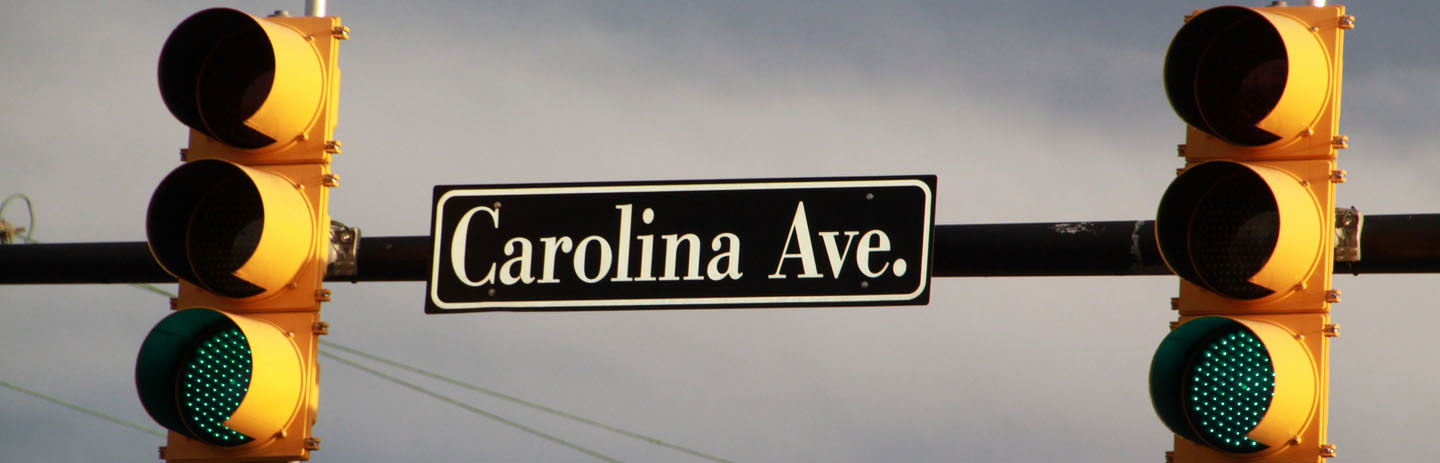The image depicts a pair of yellow traffic lights mounted on a horizontal black bar. Both traffic lights, situated on the left and right ends of the bar, are illuminated green, signaling "GO." Positioned centrally between the lights is a small black sign with white lettering that reads "Carolina Ave." The background features a cloudy, gray sky with some cloud cover, giving the scene a rather gloomy appearance. Additionally, power lines run from the left side of the image towards the center, partially obscuring the view. At the far left of the background, there is a small object that might be a bird, although it is not clearly identifiable.